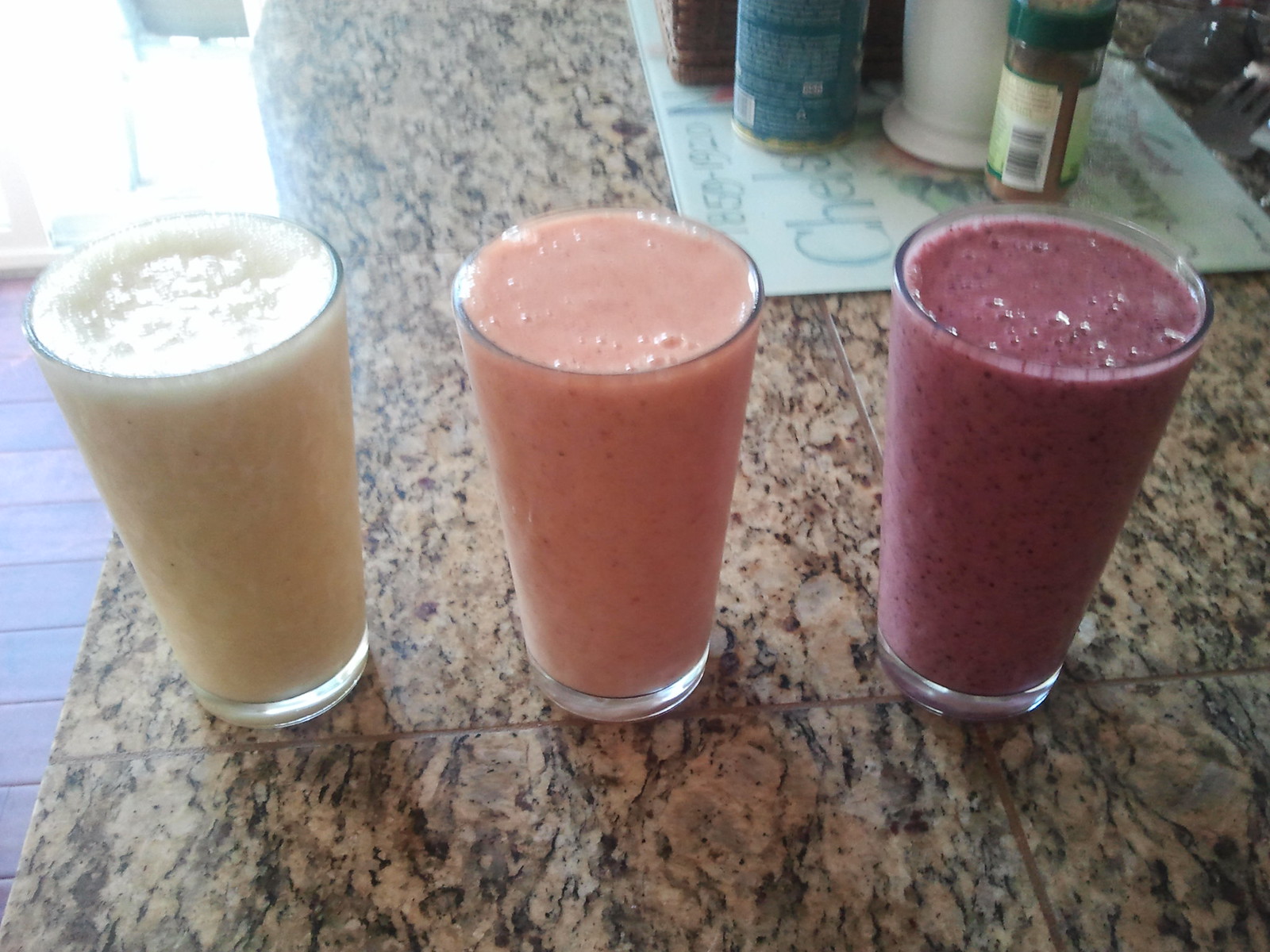This color photograph captures an indoor kitchen scene centered around a brown and black granite countertop. On the countertop, there are three tall glasses, each filled to the brim with a thick, smoothie-like beverage. The glass on the left contains a white drink, possibly a vanilla milkshake or protein drink with a slightly foamy top. The middle glass holds a vibrant pink beverage, likely strawberry-flavored. The final glass on the right is filled with a dark purple liquid, suggesting a blueberry flavor. Behind the glasses, a collection of plastic spice bottles sits on a white placemat or decorative paper. The kitchen setting also includes a glimpse of a tile floor and a well-lit window to the left, while a sign with illegible writing appears behind the countertop. The image does not feature any people or animals.